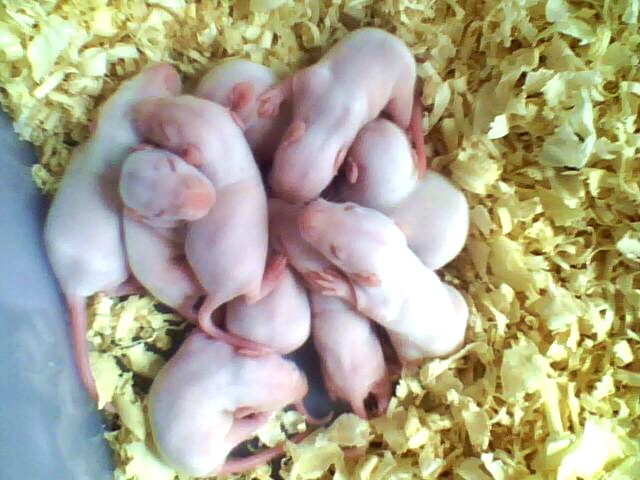This color photograph captures a large pile of tiny, pale pink baby rodents, which appear to be rats or mice, piled on top of each other towards the left and center of the image. The baby rodents, numbering at least ten, and possibly more beneath the visible pile, have closed eyes that look like dark pink slits, and their small pink noses and legs are prominently visible. They are lying on a yellow-green bedding that resembles shredded paper or mulch, commonly seen in pet stores. A blue triangular shape in the bottom left corner suggests the edge of a box or barrier containing the animals, illuminated by a soft light from above. The babies, still hairless, give the impression of cuddling together for warmth and security.